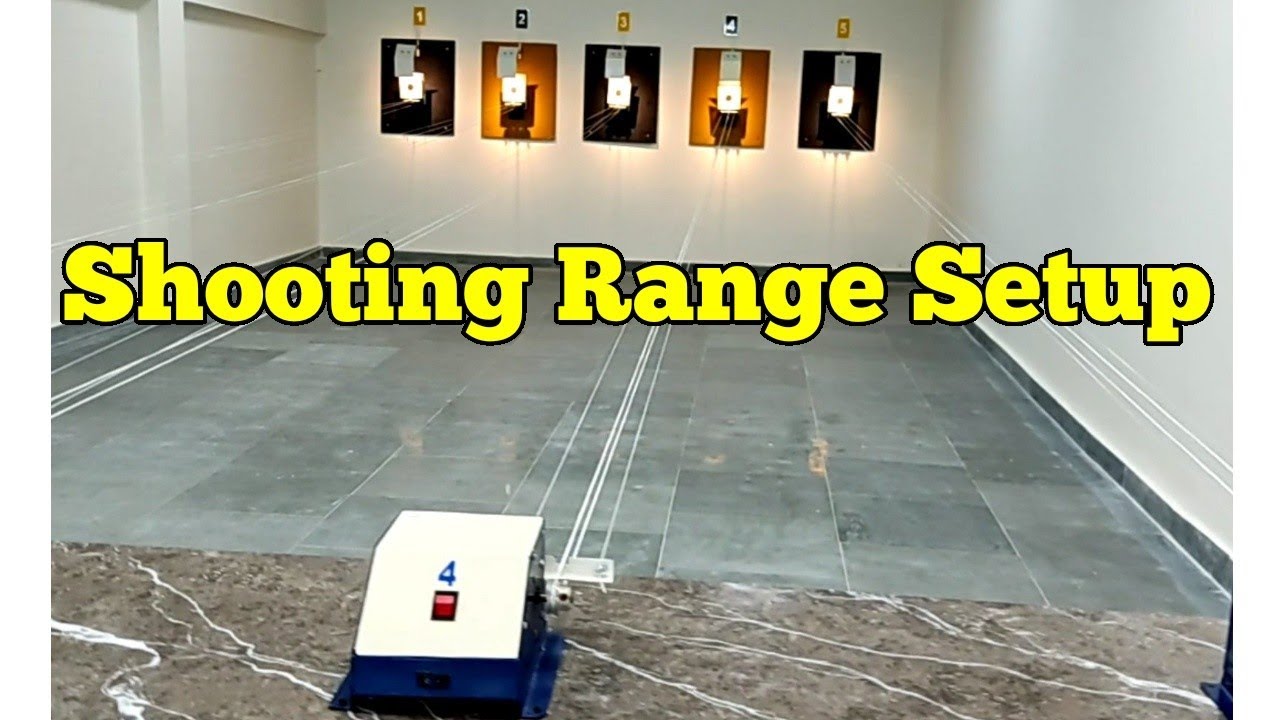The image depicts an indoor shooting range with an upscale ambiance, suggested by its gray marble-tiled floor. The room features whitewashed walls, and at the far end, multiple targets are aligned. These targets are distinguished by alternating brown and orange numbered squares, each containing a smaller white square with a red dot. Wires run from the targets toward the front of the room, connecting to white and blue devices on the floor. The scene is well-lit, emphasizing the clean, high-end setup. Dominating the image is a bold caption in large yellow letters with a black outline that reads, "Shooting Range Setup," suggesting it could be a thumbnail for a YouTube video. Overall, the shooting range is devoid of people, highlighting a pristine, ready-for-use setup.